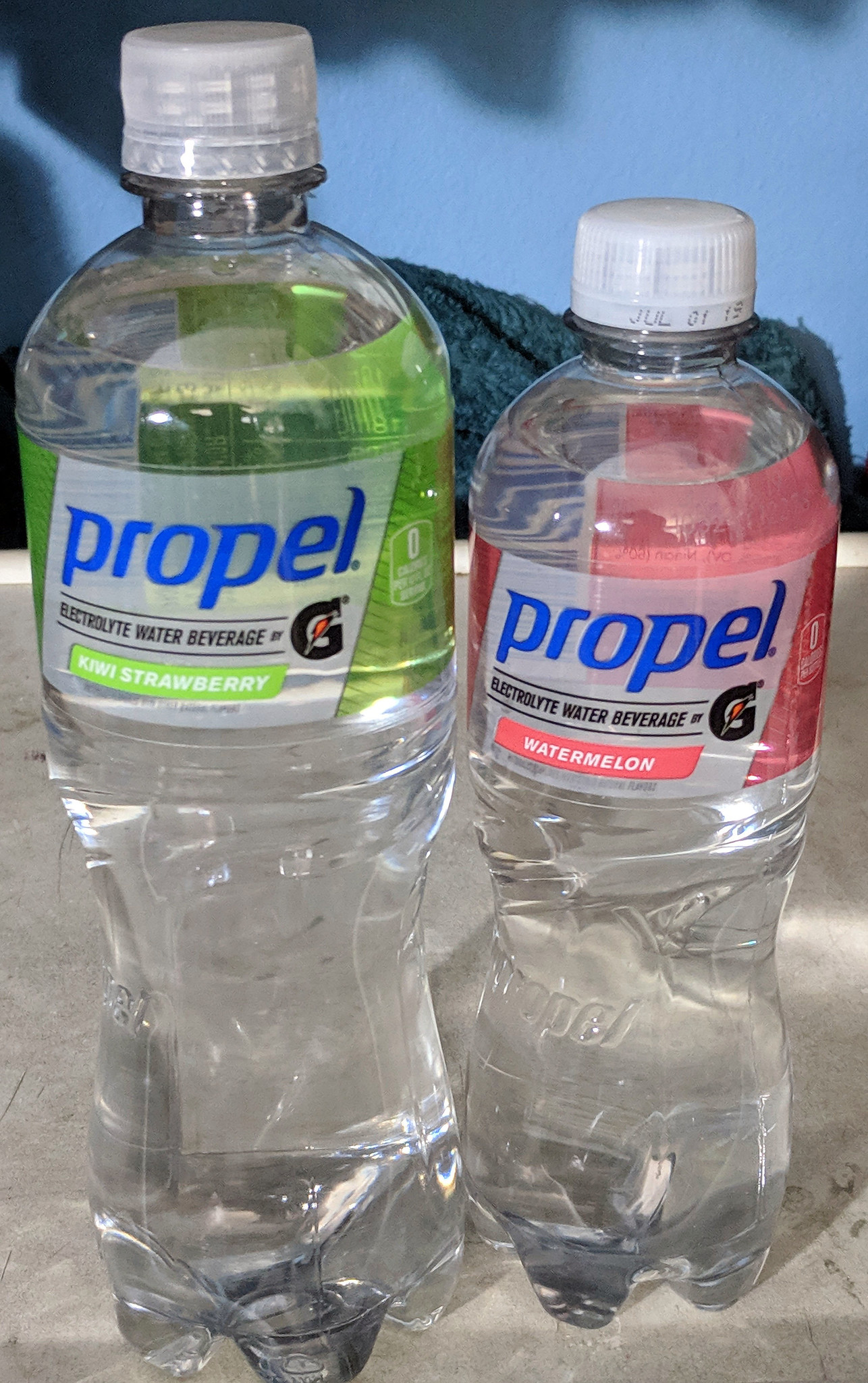In the image, two water bottles sit side by side on a scratched, light gray surface. The larger bottle on the left features a label with "PROPEL" in bold blue letters wrapping around the top half, beneath which the text "ELECTROLYTE WATER BEVERAGE" appears in black. A black line separates this from a Gatorade symbol positioned to the right. Below this, another black line precedes a neon green banner with the words "KIWI STRAWBERRY" in white text. The bottle contains clear liquid. To the right of this bottle is a smaller, nearly identical bottle. It also has a blue "PROPEL" logo, the same black text "ELECTROLYTE WATER BEVERAGE" and Gatorade symbol, but the banner is pink with "WATERMELON" written in white. Towards the bottom of each bottle, an embossed "PROPEL" logo is visible in the plastic. The background features a blue wall with some fabric draped over what appears to be the back of a chair.